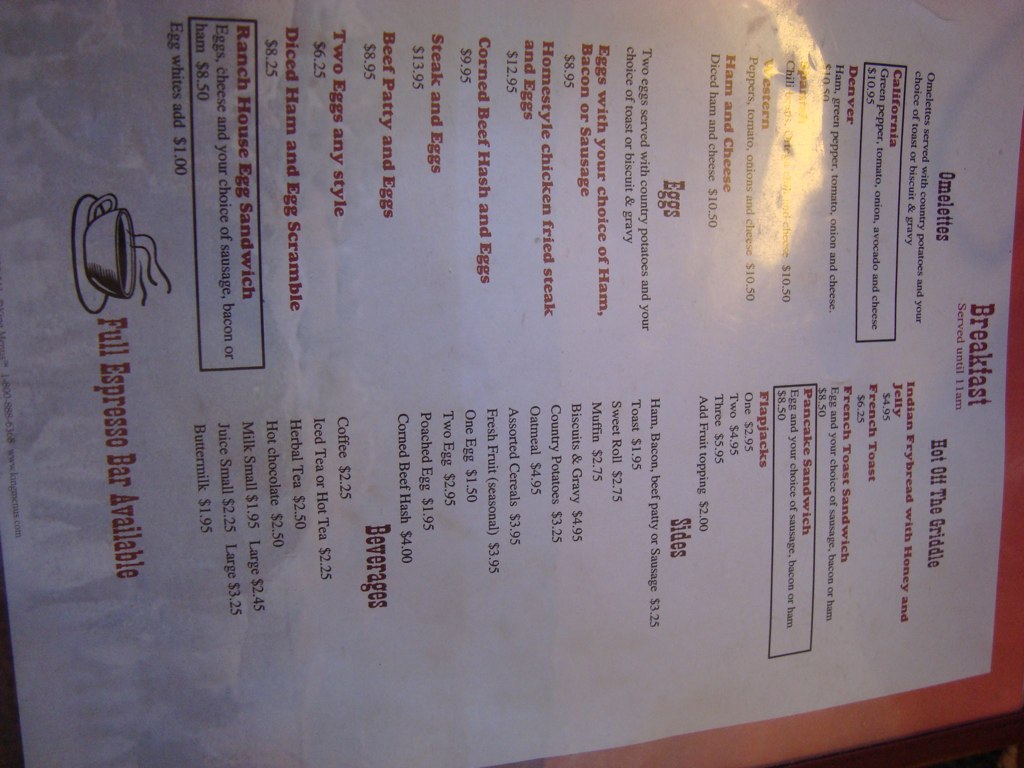This image showcases a landscape-oriented photograph of a breakfast menu, which is rotated 90 degrees from its original portrait format. The menu is likely printed on a standard 8.5 x 11-inch sheet and is laminated. It features a clean white background with text in contrasting colors: red for the headings and dish names, and black for the descriptions and prices.

"Breakfast" is prominently written at the top in red, while the bottom of the menu highlights in red text that a "Full Espresso Bar" is available. The menu is divided into categories, with "Omelets and Eggs" on the left side and "Eat off the Griddle," "Sides," and "Beverages" on the right side. Dish names such as various omelets, pancakes, and waffles stand out in red, while their descriptions and corresponding prices are in black.

Among the egg items, prices range from $6.25 for two eggs in any style to $12.95 for a homestyle chicken-fried steak and eggs. The sides are listed to include options like sweet rolls, muffins, biscuits and gravy, and country potatoes. Overall, it is a standard American breakfast menu, offering a variety of traditional breakfast dishes.